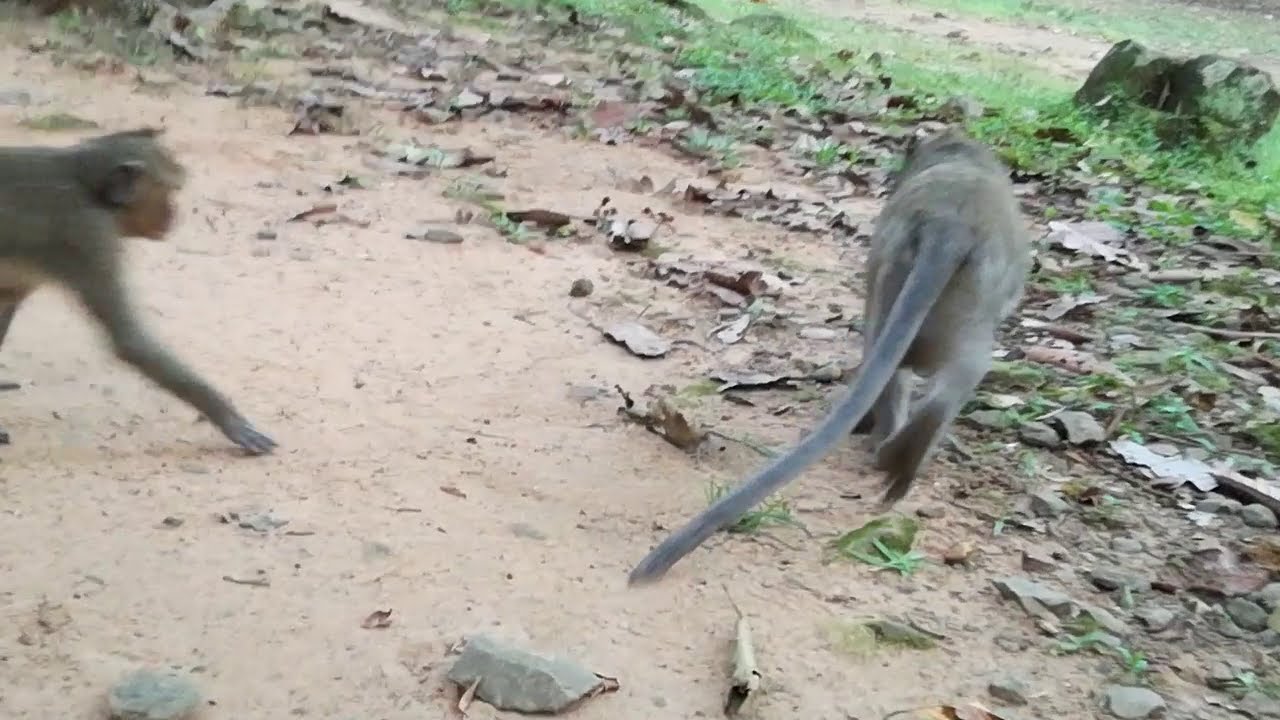This detailed outdoor image captures a natural setting that might be a part of a zoo exhibit. The foreground features a dirt ground scattered with dead leaves, a few rocks, and patches of green grass stretching towards the back. Dominating the scene are two monkeys. The monkey on the right has its back turned to the camera, showcasing a long, trailing tail and a brownish-gray coat. Its motion is captured slightly blur, indicating it's either walking or prancing away. On the left side of the frame, another monkey appears from the midsection onward, displaying its head, prominent right ear, and an outstretched right front paw in mid-motion, suggesting it's walking towards the other monkey. Both monkeys seem to be engaged in some form of activity or interaction, adding a dynamic element to the otherwise tranquil scene.